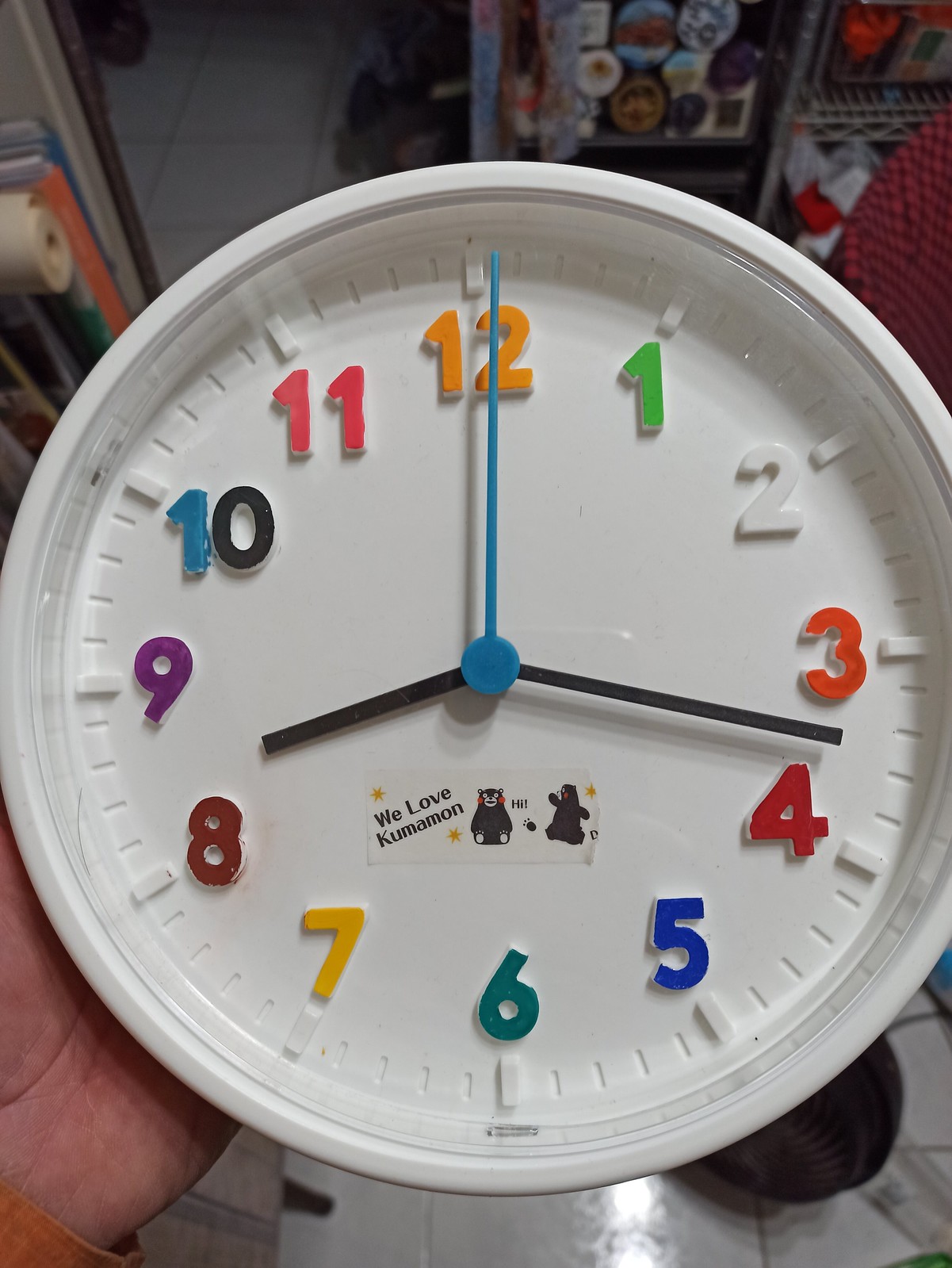In this image, we see a well-organized, mostly gray room filled with various large bundles of materials. Prominent among them are several large rolls of fabric, notably in red, blue, and white with red patterns. These rolls appear to be stored in a substantial cabinet, which neatly houses numerous rolls of different textiles. Below this cabinet, there's a pristine, white, glossy table, where a hand wearing an orange sleeve is visible. Dominating the table's surface is an adorable children's clock, constructed from shiny white plastic. This cheerful clock features multicolored numbers - green, white, orange, red, blue, purple, black, and pink - adding a playful splash of color to the room. Of its three hands, one stands out in blue while the other two are black. Additionally, a small sticker embellishes the clock, depicting the front and back of a teddy bear with a cute message that seems to read "We Love Kiss, Kiss Marison" or something similar.